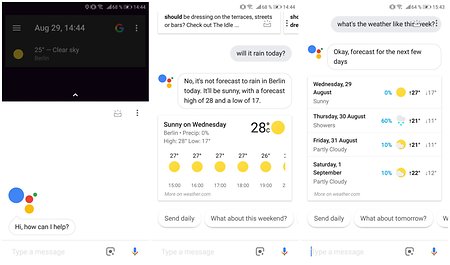"Three screenshots from the Hello Google (or possibly Google AI) app are displayed. The leftmost screenshot features a time and weather widget on a black background, indicating the date as August 29th and the time as 14:44. Below the time, the weather is shown as 25 degrees Celsius and clear skies. The Google logo is positioned in the lower left corner, accompanied by the prompt, 'Hi, how can I help you?'

The center screenshot depicts another weather interface, displaying 28 degrees Celsius and sunny for Wednesday, along with a four or five-day forecast, although the text is too small to discern specific details.

The rightmost screenshot shows an AI chat conversation where the user has asked about the weather forecast for the last week. The AI responds with the forecast for the next three days, but again, the text is too small to read specific details."